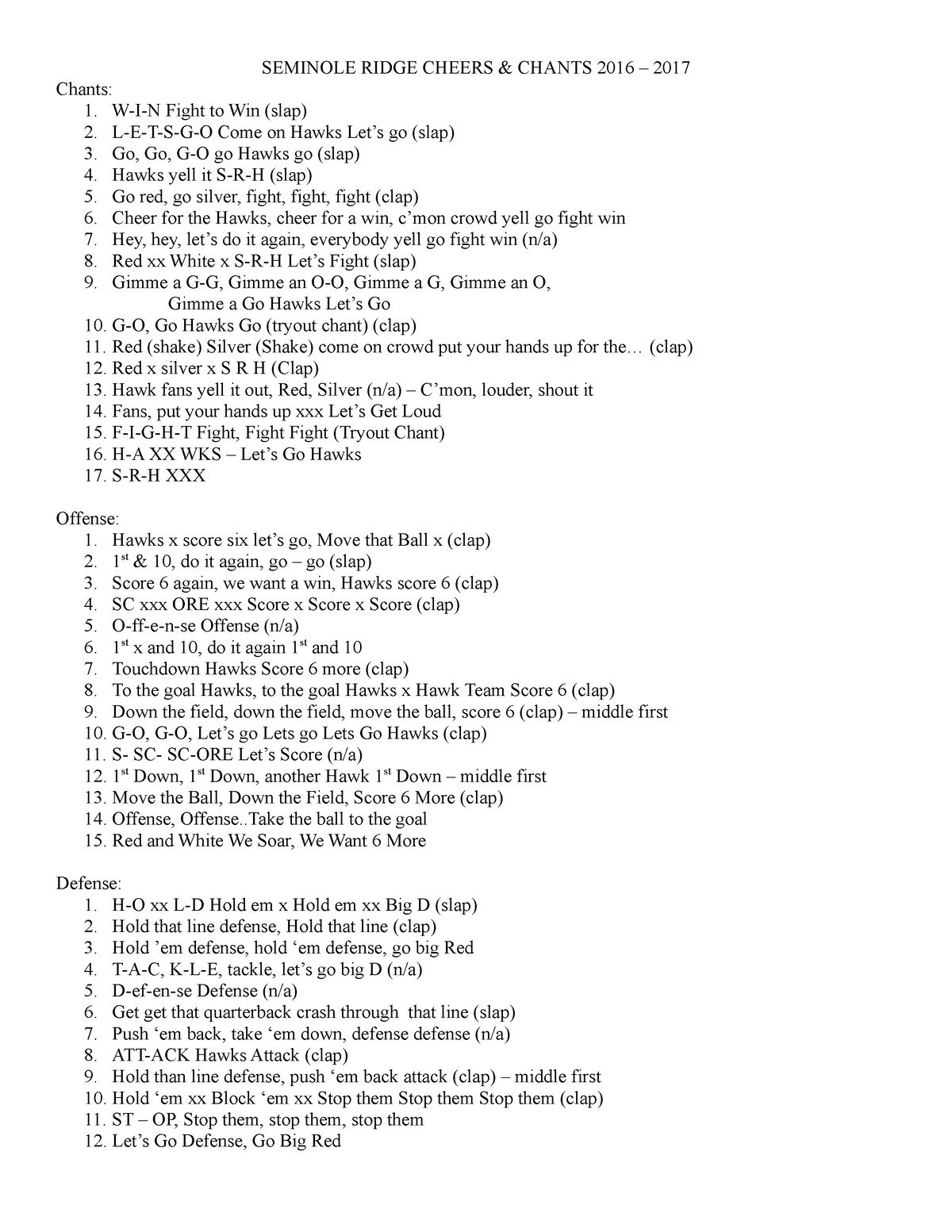The image displays a detailed list of cheers and chants designated for the Seminole Ridge cheer team for the 2016-2017 season. The content is organized into three distinct sections:

1. **Chants**: This section features 17 different chants. For instance:
    - **Number 1**: "W.I.N. Fight to Win Clap."
    - **Number 14**: "Fans, put your hands up. Let's get loud."

2. **Offense**: This section comprises 15 chants aimed at boosting the team's offensive play. Highlights include:
    - **Number 9**: "Down the field, down the field. Move the ball, score six. Clap."

3. **Defense**: This section lists 12 defensive cheers, such as:
    - **Number 3**: "Hold 'em defense, hold 'em defense. Go Big Red."

Each chant is accompanied by specific instructions, including when to spell out words, when to simply say them, and when to incorporate actions like clapping. The structured layout indicates clear directions for cheerleaders, ensuring synchronized and spirited performances during games. The list demonstrates a well-thought-out strategy to maintain crowd engagement and team morale through organized cheer routines.